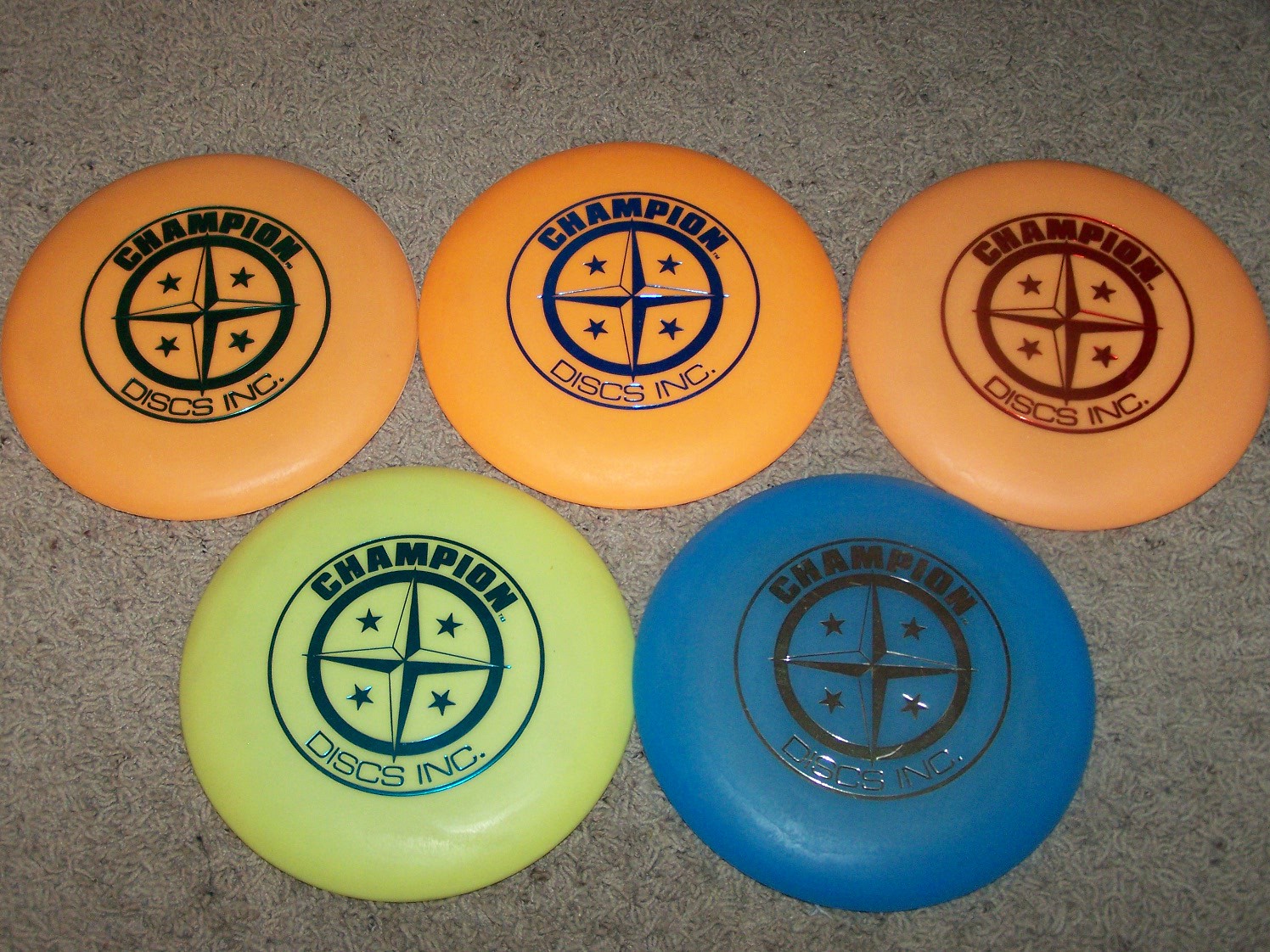The image displays five disc golf frisbees arranged on a slightly dirty, neutral tan carpet. Each frisbee features the same logo from Champion Discs Inc., with a central 4-pointed star surrounded by four small 5-pointed stars and the text "Champion" at the top and "Discs, Inc." at the bottom of the circle. There are three shades of orange frisbees: two have a pale or dusty orange hue, while one is a bright, shiny orange. The remaining two frisbees are bright yellow and royal blue. The writing's color on all the discs varies—black on one orange, yellow, and blue frisbee, blue on another orange frisbee, and red on the last orange frisbee. These frisbees, all of standard size and shape, are lined up with three on top and two at the bottom, touching and uniformly aligned.